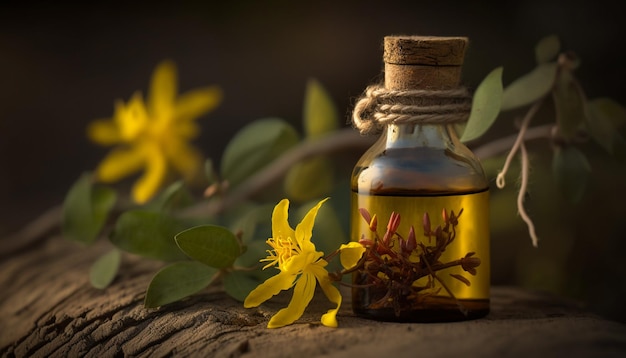In this color photograph of realistic product photography, the subject is a small bottle of greenish oil, possibly essential or olive oil, positioned on the right side of the landscape-oriented image. The bottle has a short, rounded bottom with a tapered neck, capped with a flat cork stopper. Beige twine is wrapped several times around the neck of the bottle, enhancing its rustic appeal. Inside the oil, flower sprigs add a delicate touch.

The bottle sits on a dark wooden surface, visible with subtle grain and texture, which slopes gently to the left. In front of the bottle, a yellow flower blossom with six slender petals and a cluster of yellow stamens occupies the bottom center of the image. The background, primarily black but blurred and out of focus, hints at another yellow flower and dark green leaves, which are tapered at both ends and add depth to the scene. The contrasting colors and textures between the vibrant yellow flowers, dark green leaves, and rustic wooden surface create a visually intricate composition emblematic of representational realism.